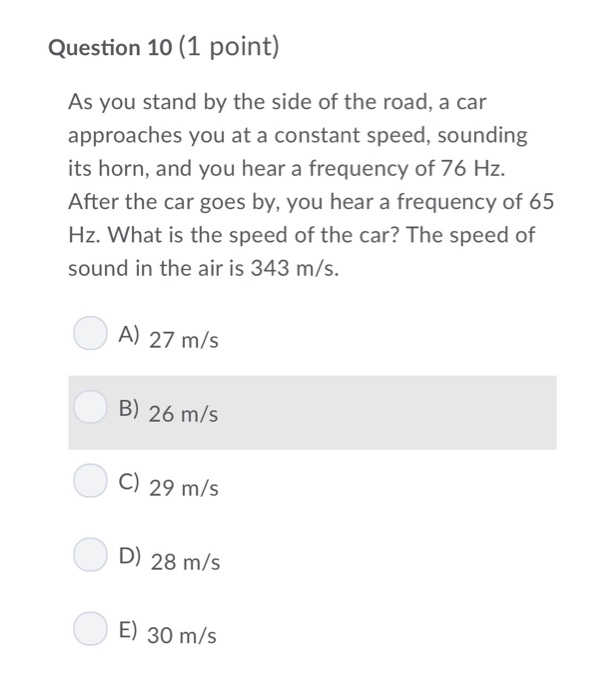The image features a white background with a multiple-choice question displayed prominently at the top left in slightly bolded black lettering. The text reads: 

"Question 10 (1 point)"

Approximately one inch below this heading, the problem statement begins with a capital "A," reading:

"As you stand by the side of the road, a car approaches you at a constant speed, sounding its horn, and you hear a frequency of 76 Hz. After the car goes by, you hear a frequency of 65 Hz. What is the speed of the car? The speed of sound in the air is 343 m/s."

Beneath this text, five answer options are presented, each prefaced by a light gray circle. The options are highlighted in alternating styles:

- **A) 27 m/s** (with a light gray circle to the left)
- **B) 26 m/s** (enclosed in a gray rectangle, with a light gray circle to the left)
- **C) 29 m/s** (with a light gray circle to the left)
- **D) 28 m/s** (with a light gray circle to the left)
- **E) 30 m/s** (with a light gray circle to the left)

The entire document maintains a clean, minimalist design focused on clarity and readability.